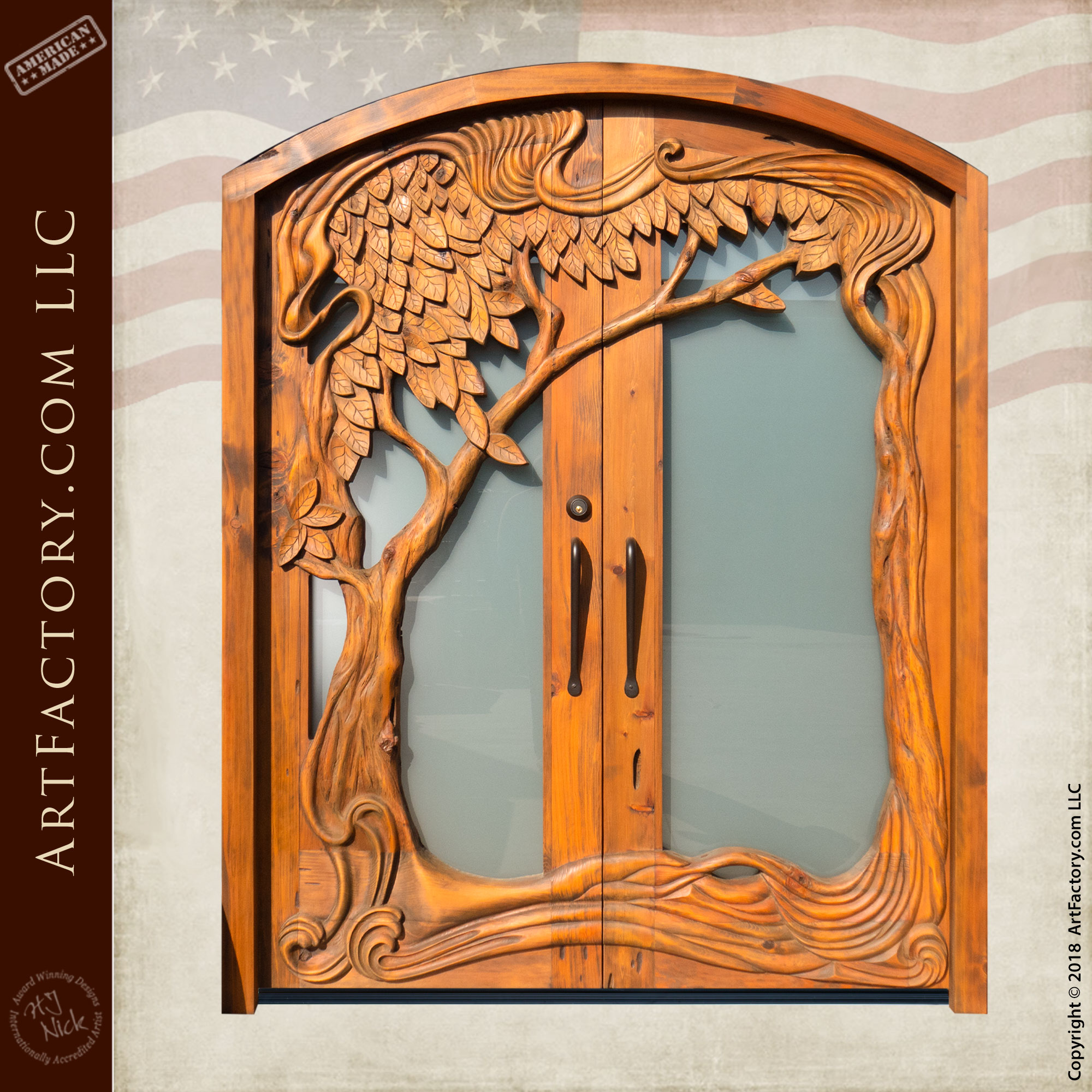The image features a large, vertical brown strip on the left-hand side with the text "Artifactory.com, LLC, American-Made" displayed prominently. Below this text is a circular logo with the letters "HG Nick" in yellow and the phrase "American Made" in gray. The background of the image is predominantly gray with a very faded and blurred American flag at the top, where the red stripes and blue field appear almost gray. 

Centrally positioned in the image is an ornate, arch-style doorway with swinging doors made from a light to medium orange-brown wood. These doors feature delicately carved tree designs, with branches and roots extending across the glass panels. Each door has a black handle and a lock positioned above the handles. The glass panes behind the carved wooden designs are opaque, adding to the intricate and decorative appearance of the doorway. Additionally, the bottom right corner of the image includes a footnote that reads "© 2018 Artifactory.com, LLC."